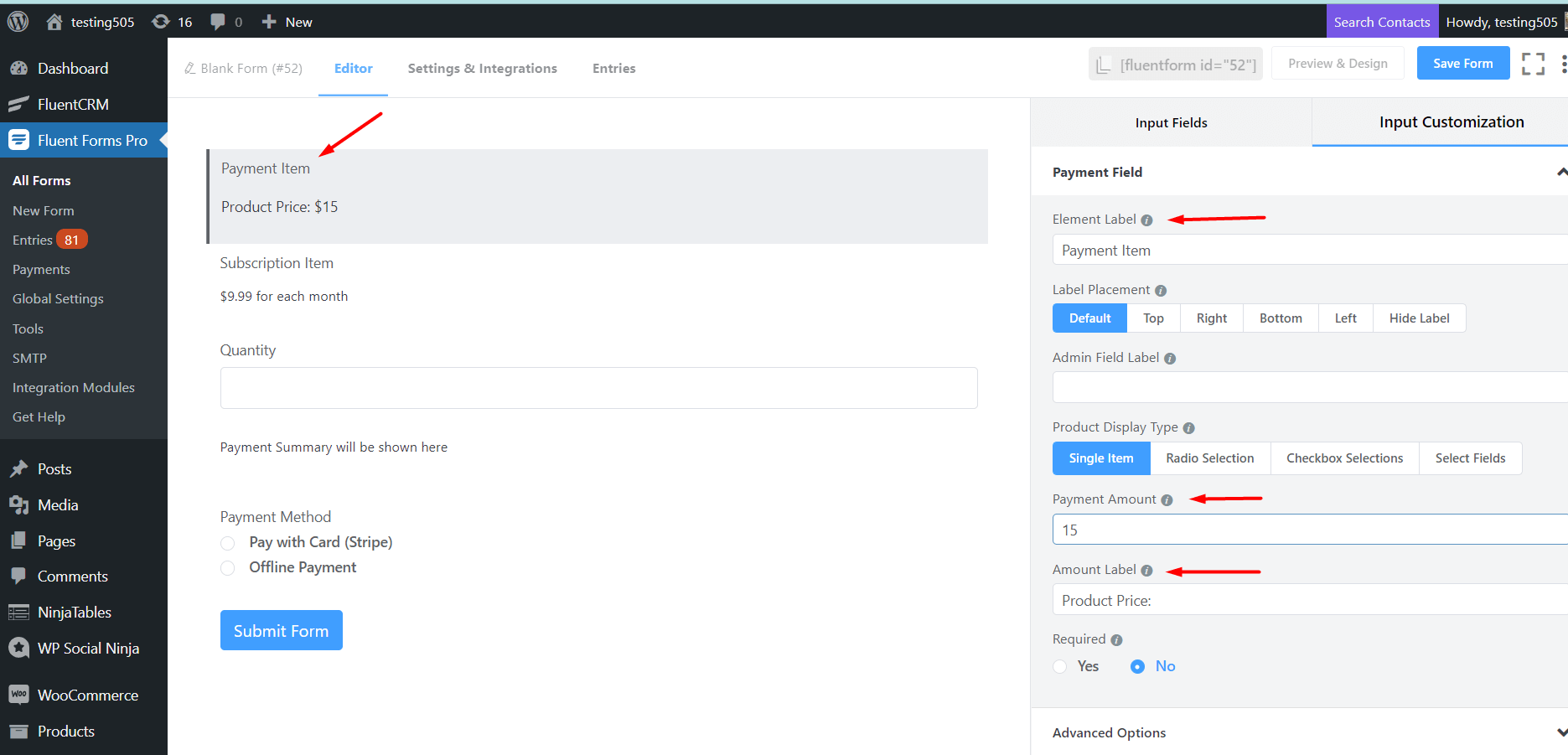In the image, a program window is open in the background, displaying the "Radar" page with the header "Testing 505" located at the top left corner, next to a W logo and a home screen icon. The dashboard features a comprehensive menu with options including Fluent CRM, Fluent Forms Pro, All Forms, New Forms, Entries (with 81 notifications), Payments, Global Settings, Tools, SMTP, Integration Modules, Get Help, Posts, Media, Pages, Comments, Ninja Tables, WP Social Ninja, WooCommerce, Products, Blank Form, Editor, Settings and Integrations, and Entries. An arrow points towards the "Payment" item, indicating that the product price is $15, while a subscription item is priced at $9.99 per month. At the bottom of the page, there are options to submit the form and choose a payment method, including card payment, Stripe, or offline payments.